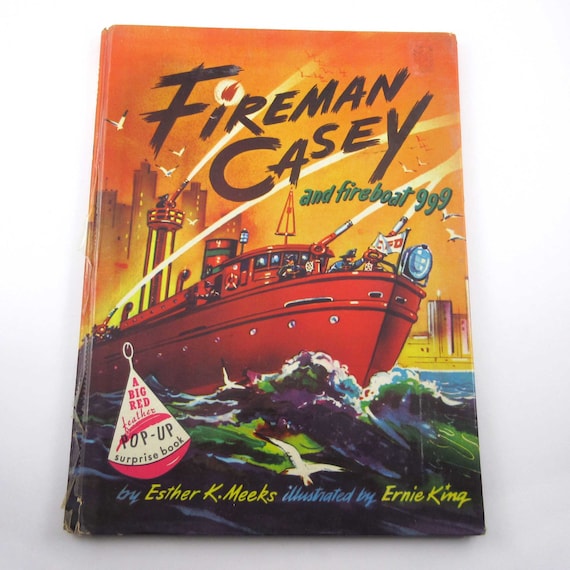The photo shows the worn cover of the hardcover book "Fireman Casey and Fireboat 999," which appears old with plastic seams coming off the binding. The cover is set in a dramatic cityscape backdrop with orange and yellow hues, giving the impression of a fiery sky. The bright red fireboat, Fireboat 999, is navigating through wild, colorful waves in shades of blue, purple, and green. The illustrated firefighters, wearing flat-brimmed black hats, are on deck, operating at least four water cannons aimed at the fiery scene, with two seagulls visible above. The title "Fireman Casey" is rendered in black, paintbrush-like font, and below it, "and Fireboat 999" is in green. A white and pink buoy is visible on the bottom left corner with the text “A Big Red Feather Pop-Up Surprise Book.” The book is credited to author Esther K. Meeks and illustrator Ernie King, with their names highlighted in blue and yellow at the bottom.